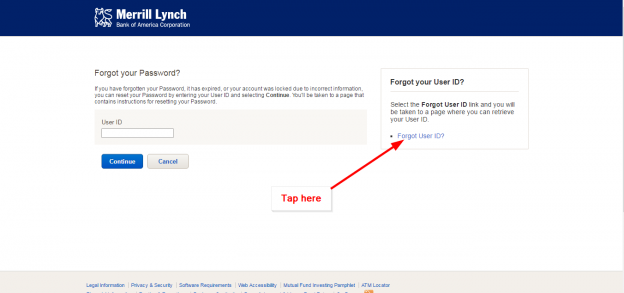On the financial services website of Merrill Lynch, the page displayed is for users who need to recover their forgotten passwords. At the top, a thick dark blue banner prominently features the Merrill Lynch logo, alongside the name "Merrill Lynch" and the phrase "A Bank of America Corporation" in smaller print.

Below this banner, the page transitions to a clean, white background. Centered at the top of this portion is the bold text "Forgot Your Password?" followed by a question mark. Beneath this heading are instructions guiding users to input their user ID.

Directly below the instructions, there's a text box where users can enter their user IDs. After filling in the ID, users can choose between two options: "Continue" to proceed with the password recovery process or "Cancel" to abort the operation.

On the right-hand side of the page, there are additional instructions for users who have also forgotten their user IDs. It explains that by selecting the "Forgot Your User ID" option, users can navigate to a specific page dedicated to retrieving user IDs. A red arrow points to this option, with a noticeable "Tap Here" label directing users to the appropriate action.

At the very bottom of the page, a gray bar contains small text that is difficult to read due to its size. This text likely includes additional information or disclaimers pertinent to the page's functionality.